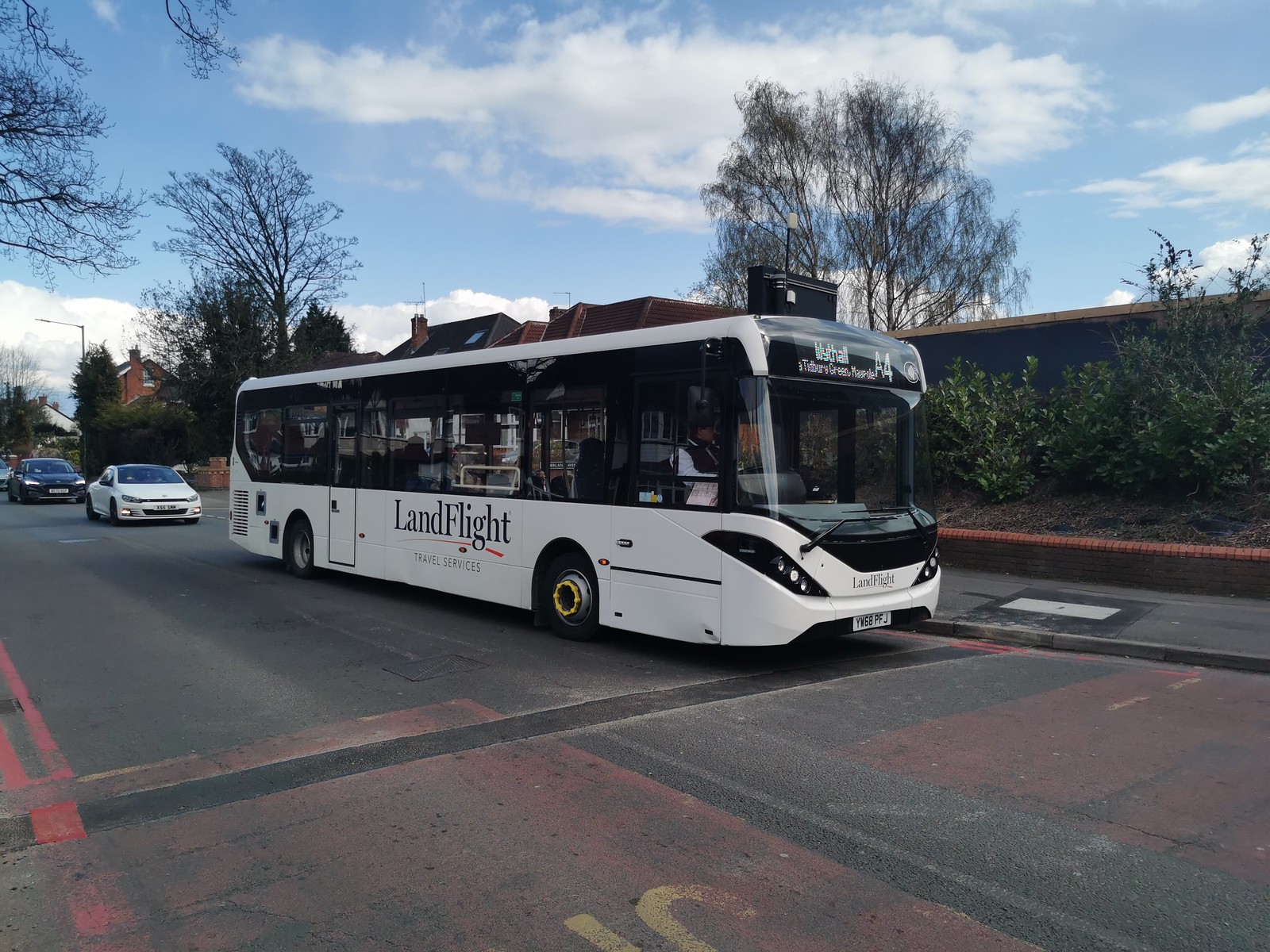The photograph captures a detailed cityscape scene featuring a large white bus with "Land Flight Travel Services" prominently displayed on its side. The bus, characterized by its predominantly windowed upper half, is moving along a street paved with dark asphalt and irregular red paint markings. The digital display at the front of the bus reads "Y Hall, A4," and beneath the windshield, it is marked with "Land Flight, YM68PFJ." Inside the bus, passengers and a bus driver are visible. Following the bus on the street are two small sedans, one white and the other black. In the background, there is a sidewalk adjacent to the bus, flanked by a raised wall covered with green-leafed bushes. Further back, a mix of houses, office buildings, and trees paint the landscape. The sky above is clear and blue, adorned with wisps of white clouds, suggesting a bright daytime setting. The image is rendered in a realistic photographic style, capturing every element in vibrant detail.